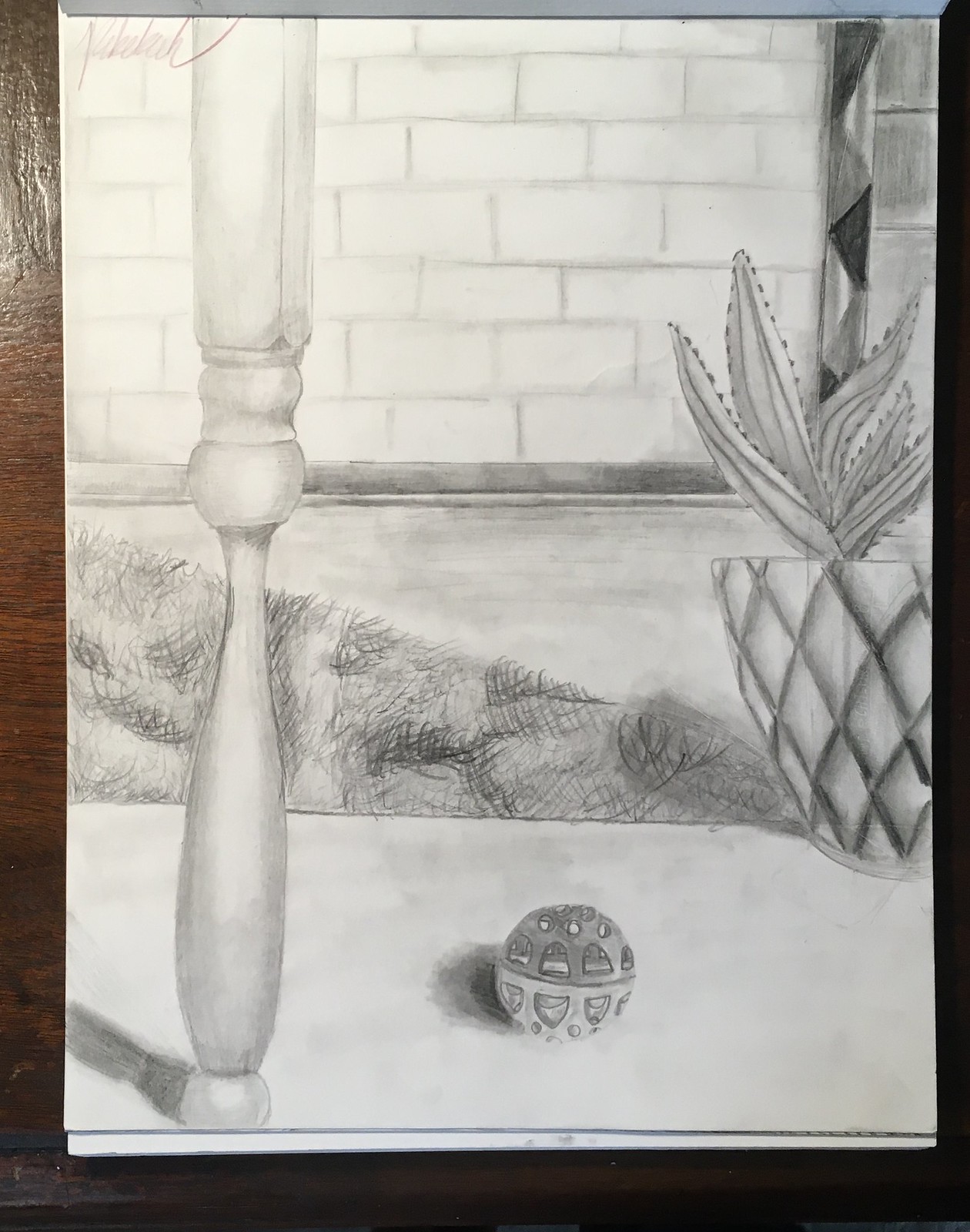A finely detailed pencil sketch displayed on a piece of pristine white art paper rests on a rich, cherry wood table. The table surface is visible on the right, left, and bottom edges of the image. The sketch itself portrays an intricate scene featuring the elegantly curved leg of a Queen Anne table set in an outdoor environment. The table leg extends vertically from the bottom to the top of the paper, dominating the foreground. 

In the background, a white brick wall provides a stark but subtle contrast. To the left side of the table leg, the scene is adorned with an outdoor curtain that features a pattern of alternating triangles cascading downward. A hint of a window is visible through the curtain, adding depth to the background. At ground level, behind the table leg, a small plot of grass can be seen, enhancing the outdoor setting. Midway up on the left-hand side, a potted plant with long, leafy fronds sits in a planter decorated with a crisscross diamond pattern.

In the bottom left portion of the sketch, near the center of the image and next to the table leg, lies a small ball with multiple holes. This detail suggests it could be a wiffle ball or a toy ball for a pet or child. The entire composition, rendered in pencil, is devoid of color but rich in texture and detail, capturing the viewer’s attention with its meticulous artistry.